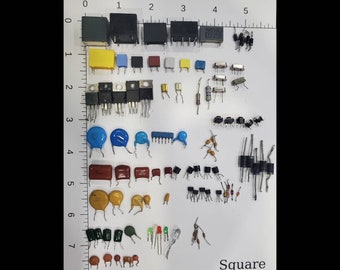The image is a detailed photograph displaying a white sheet of paper set against a black background. This sheet is marked with ruler measurements along its edges, extending from 0 to 7.5 inches vertically on the left side and from 0 to 5 inches horizontally across the top. The numbers are aligned such that they appear tilted at 90 degrees. The sheet features eight distinct rows of small electronic components, organized neatly within the central portion.

The top row consists of black and gray square components, likely electronic fuses or capacitors. Below this are rows with multicolored components, each displaying a vivid array of colors including yellow, blue, tan, red, and black. Some components are square, some are circular, with various sizes and shapes. Each of these has tiny prongs, suggesting they are parts typically used in electronic assemblies.

Towards the middle, blue circular components and tan circular ones that appear waxy are visible. The bottom-most row contains the smallest components which are red and waxy in appearance. 

Lastly, the bottom right corner of the sheet bears the watermark "Square," written in gray with a capitalized "S". The entire setup looks meticulously organized as if showcasing these components for cataloging or illustrative purposes.